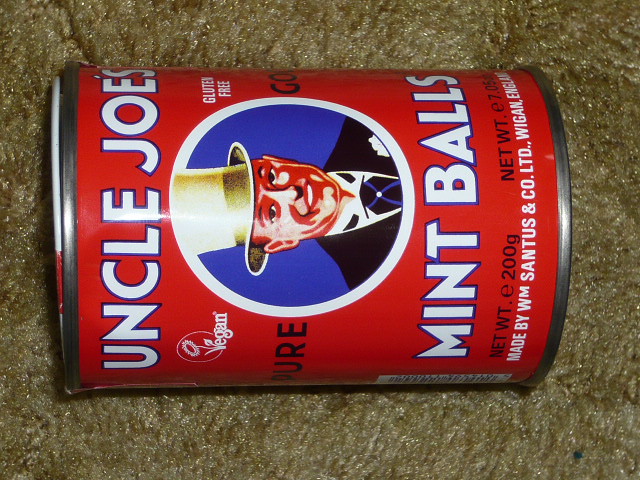This detailed, close-up photograph shows a can of Uncle Joe's Mint Balls laid on its side on a brownish carpet, filling almost the entire horizontal frame. The bottom of the red can is to the right while the top is to the left. The can features a red label with white text outlined in blue, stating "Uncle Joe's Mint Balls". Central to the design is an oval image of a white gentleman wearing a gold top hat, black tuxedo, white shirt, and a blue tie. His face has a reddish tint and he is smiling, displaying his white teeth. The label includes various texts: "Pure" to the left of the oval and "G.O" to the right. Additionally, it mentions the product as vegan and gluten-free, with the net weight being 200 grams or 7.7 ounces. Made by William Santus and Company Ltd, from Wigan, England, this can’s barcode is partially visible. The label details are meticulously printed in a combination of white, black, and blue accents, enhancing its vintage charm.